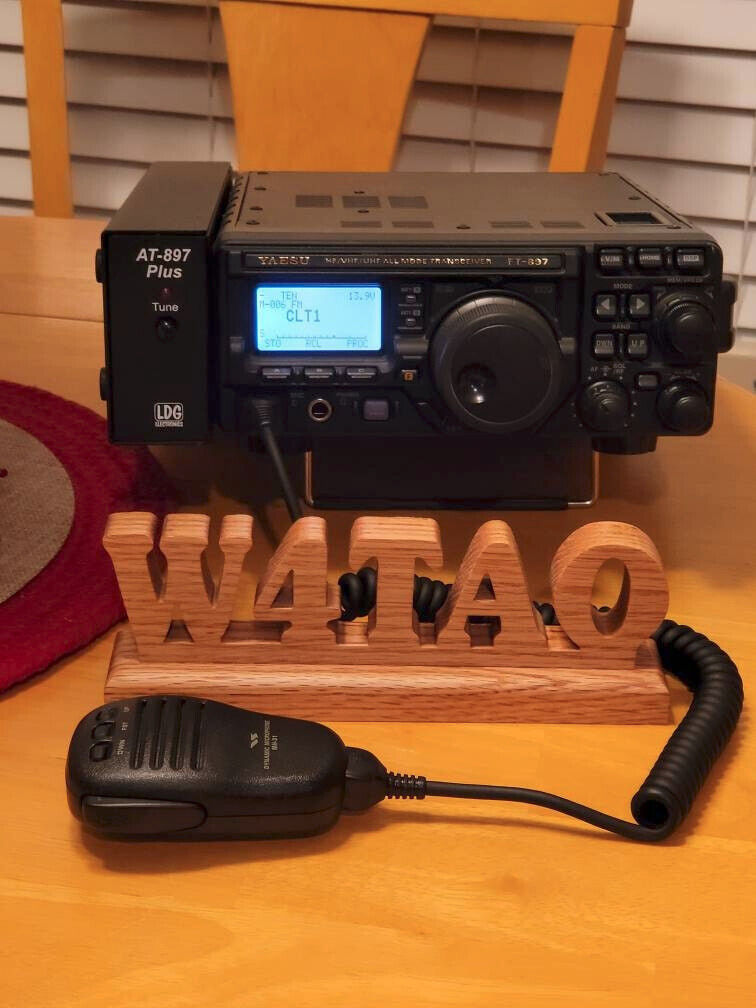The image is a detailed, portrait-oriented color photograph featuring a communications setup prominently centered on a light brown wooden table. The main subject is a black YAESU radio unit, model AT-897+, with an attached handheld elliptical-shaped black microphone connected by a coiled cord. The radio has a large black knob near its center and a blue-lit digital screen displaying "CLT1" situated towards the left-center. The top of the radio displays white text labeling the model, and "TUNE" beneath it, along with "LDG" at the bottom. Supporting the radio is a small metal arm. Positioned in front of the radio is a smooth, light-colored wooden plaque with the three-dimensional letters "W4TAO," adding a touch of craftsmanship to the scene. The background includes a partial view of a person in a brown shirt, white window blinds, and a partially visible wooden chair. The clear focus and realism of the photograph effectively capture every detail of the radio setup.